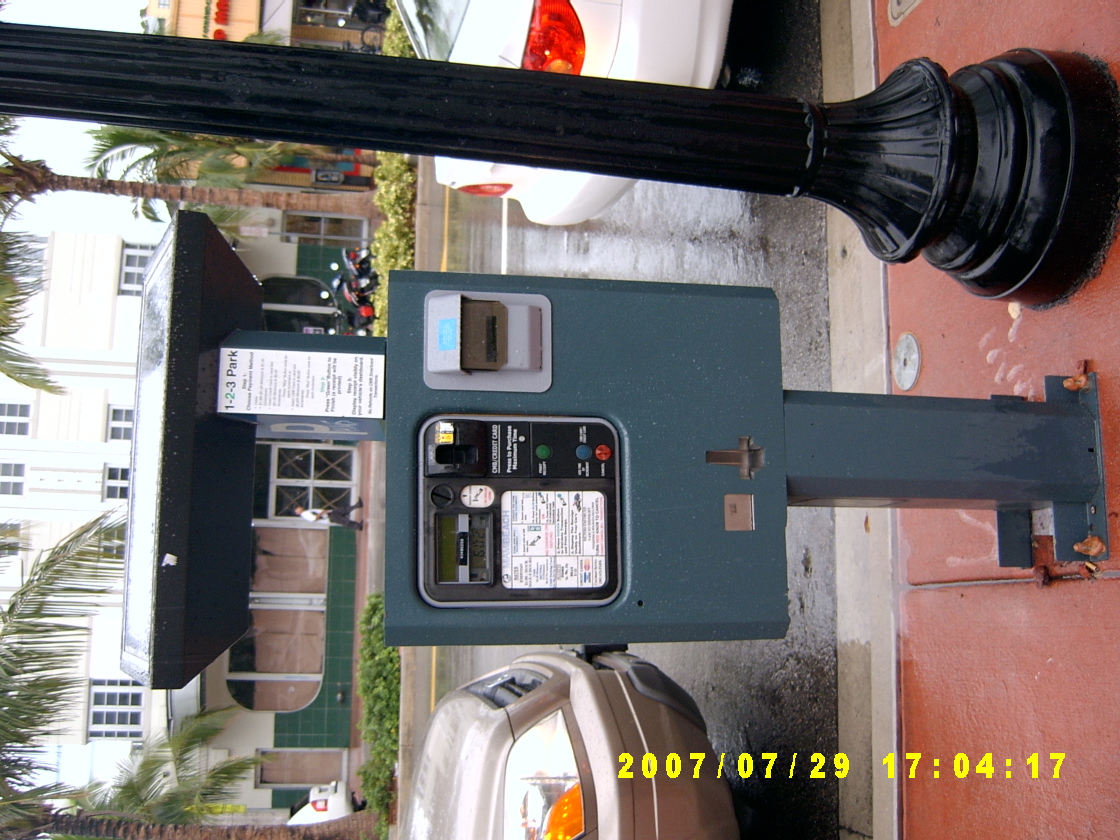This tilted horizontal image, originally a vertical photograph, captures a city street scene with a focus on a distinctive parking meter. The parking meter, prominently positioned near the center, is a teal blue, rectangular structure featuring an overhanging roof labeled "1-2-3 Park." It has both a cash slot on the right and a credit card swipe on the left, with a black and white display indicating parking charges. To the left of the parking meter stands the base of a black lamppost. The photo timestamp, "2007-07-29, 17-04-17," is displayed in thick yellow text at the bottom right corner. Nearby, the street is black and appears wet, bordered by a red concrete sidewalk and a gray curb. Two cars are parked adjacent to the meter: a brown/tan car in the foreground and the tail-end of a white car farther back. The scene is set against a backdrop of a white building on the far left and greenery that suggests a warm climate, indicated by palm-like trees and flowers along the road.